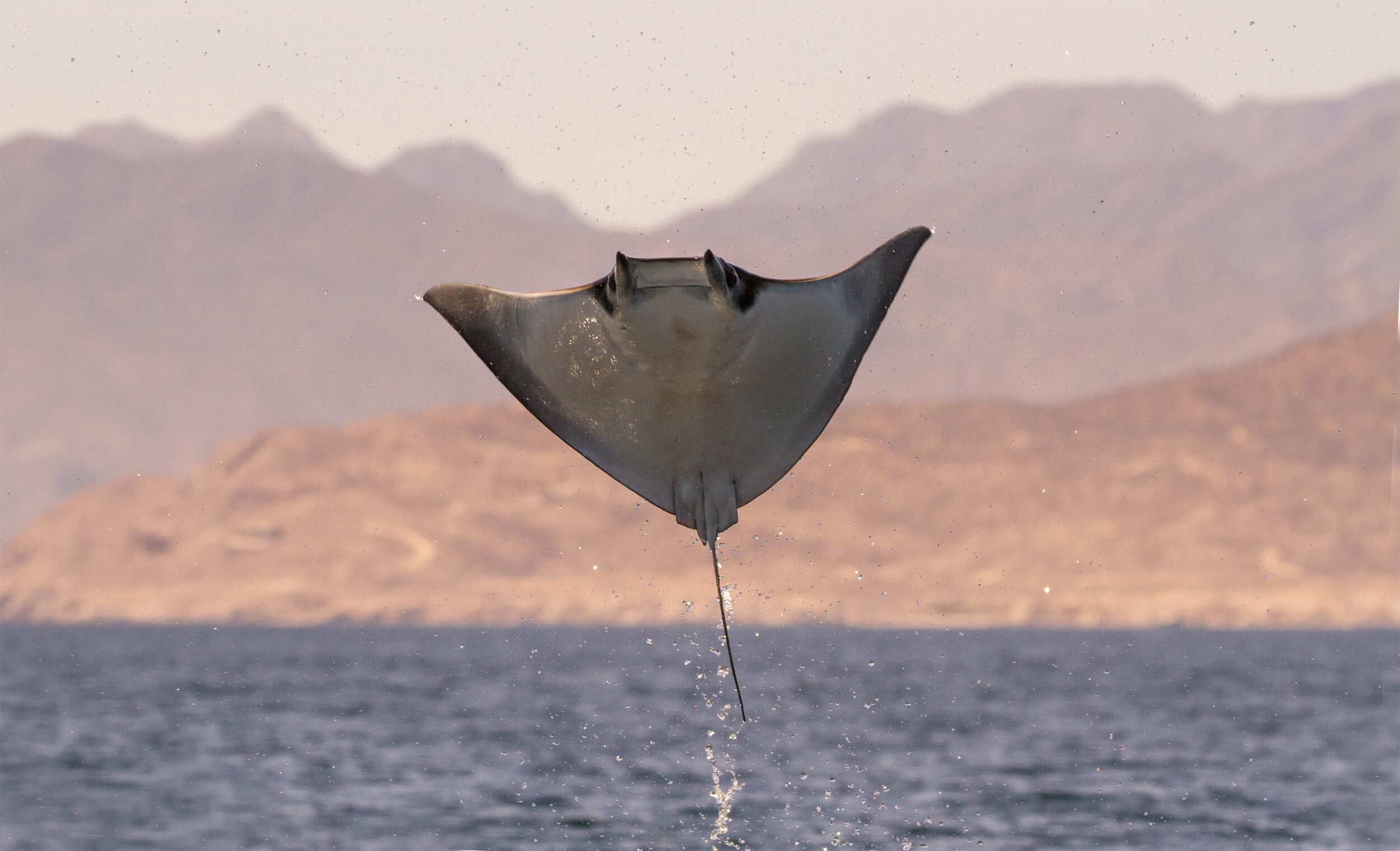In this outdoor image, a dramatic scene unfolds with a manta ray leaping gracefully out of the blue water in the foreground. The water features a mix of blue shades, accentuated by splashes of darker blue and white froth where the manta ray emerges. The creature's long, slender tail is clearly visible, along with its predominantly white underbelly. Its eyes, positioned on the sides, are a darker shade, and the tips of its fins display a darker gray hue.

Beyond the water lies a tan, dirt-like hilly area that stretches across the image, tapering off to the left. Behind this, a range of taller hills or perhaps a mountain range, slightly blurry and adding depth, rises in the distance. These hills possess a light brown to purple hue, becoming more faded towards the top of the picture. The sky above is a light gray with subtle purple undertones, creating a soft, ethereal backdrop to this striking marine moment.